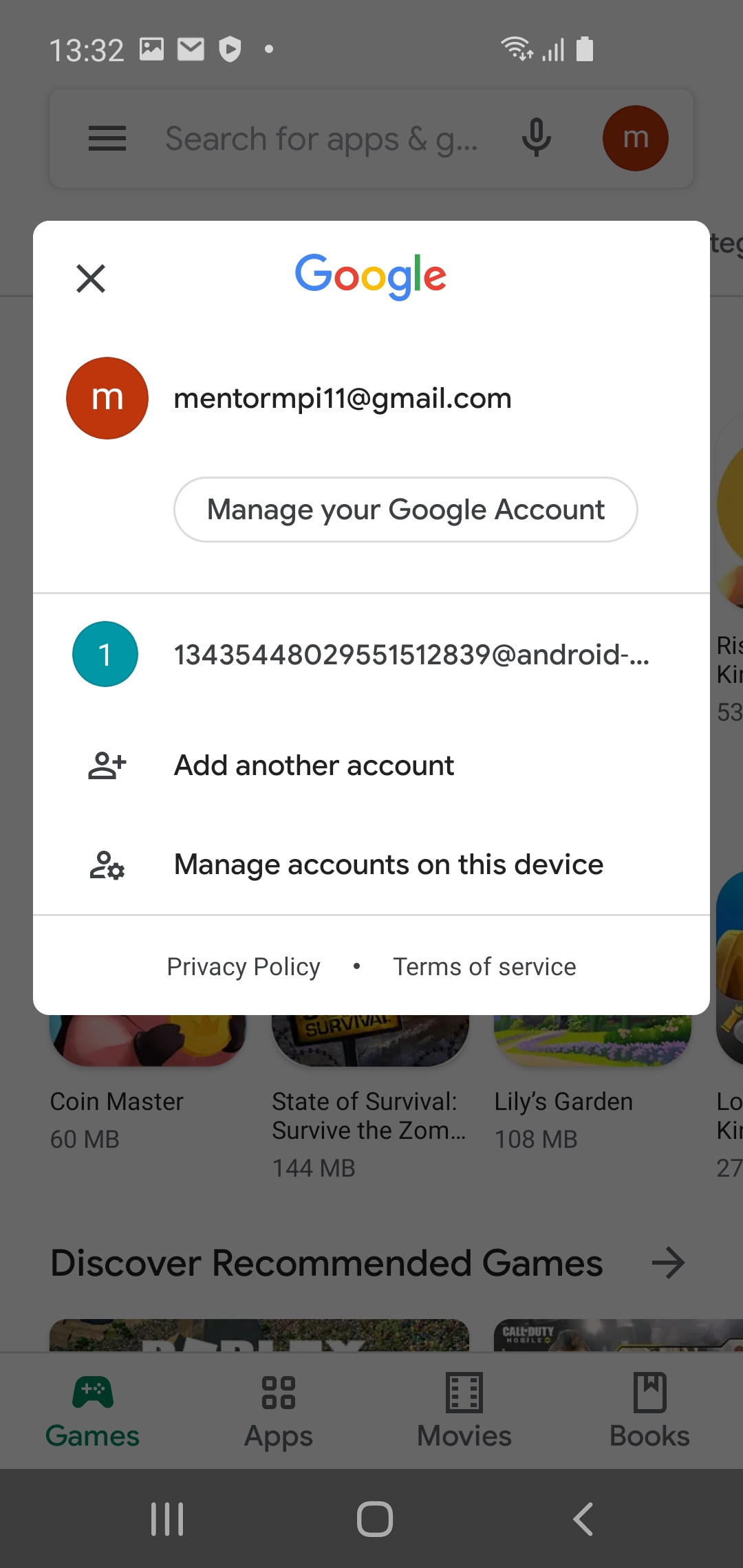Certainly! Here is a cleaned-up and highly detailed caption for the described image:

---

A mobile screenshot showcasing an interface from a Google app on a smartphone. In the background, the Google Play Store is faintly visible, displaying several app icons and names such as "Coin Master," "State of Survival," "Survive the Zombies," and "Lily's Garden," along with their respective file sizes, though some text is partially cut off. 

The focal point of the image is a white, rounded rectangular pop-up in the center featuring the Google logo at the top. Below the logo, the currently signed-in username, mentormpi11@gmail.com, is displayed prominently. An avatar appears next to the username, depicted as a rusty orange-red circle with a white letter 'M' inside. 

Directly beneath the username, a gray text button labeled "Manage your Google account" is visible. Another account linked to the device is also shown, identified by a long numerical sequence, partially cut off, suggesting it might be associated with a phone, ending with "@android-". 

The pop-up includes additional options like "Add another account" and "Manage accounts on this device," each accompanied by small icons to the left of the text. At the bottom of the pop-up, links to the "Privacy Policy" and "Terms of Service" are shown in smaller text.

---